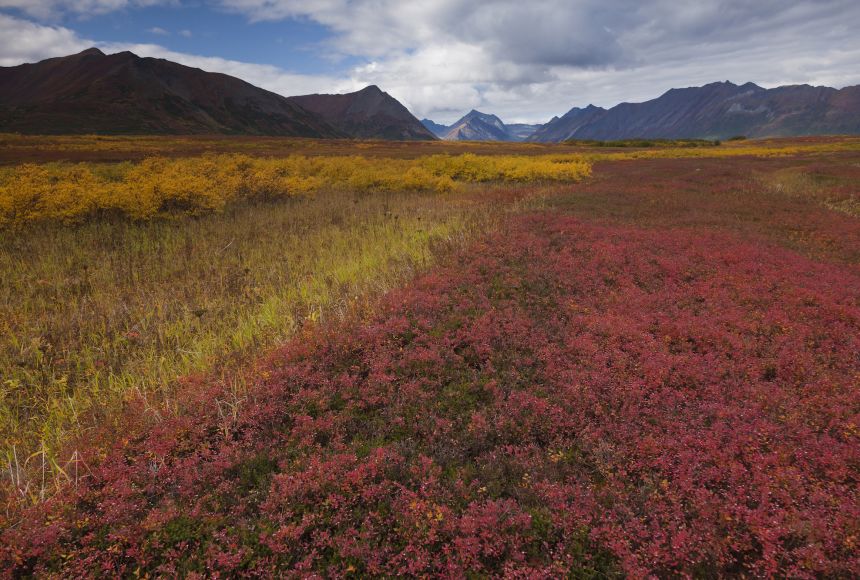This outdoor color photograph showcases a breathtaking landscape dominated by a rocky, grass-covered mountain range stretching across the background from left to right, noticeably free of snow. Above the range, the sky is partly cloudy with a patch of bright blue visible in the upper left corner, providing a striking contrast against the clouds that occupy the upper right. The expansive foreground, which makes up over 75% of the image, is a vibrant and colorful field divided into various sections of wildflowers and plants. Dominating the lower right corner are dense clusters of blooming pinkish-red wildflowers, creating a vivid splash of color. The left side of the field features tall green prairie grasses, while midway up the image near the horizon, a line of bright yellow wildflowers stretches across, resembling goldenrod. With no animals or man-made structures in sight, the scene exudes a serene and untouched natural beauty, likely reminiscent of a tranquil meadow.